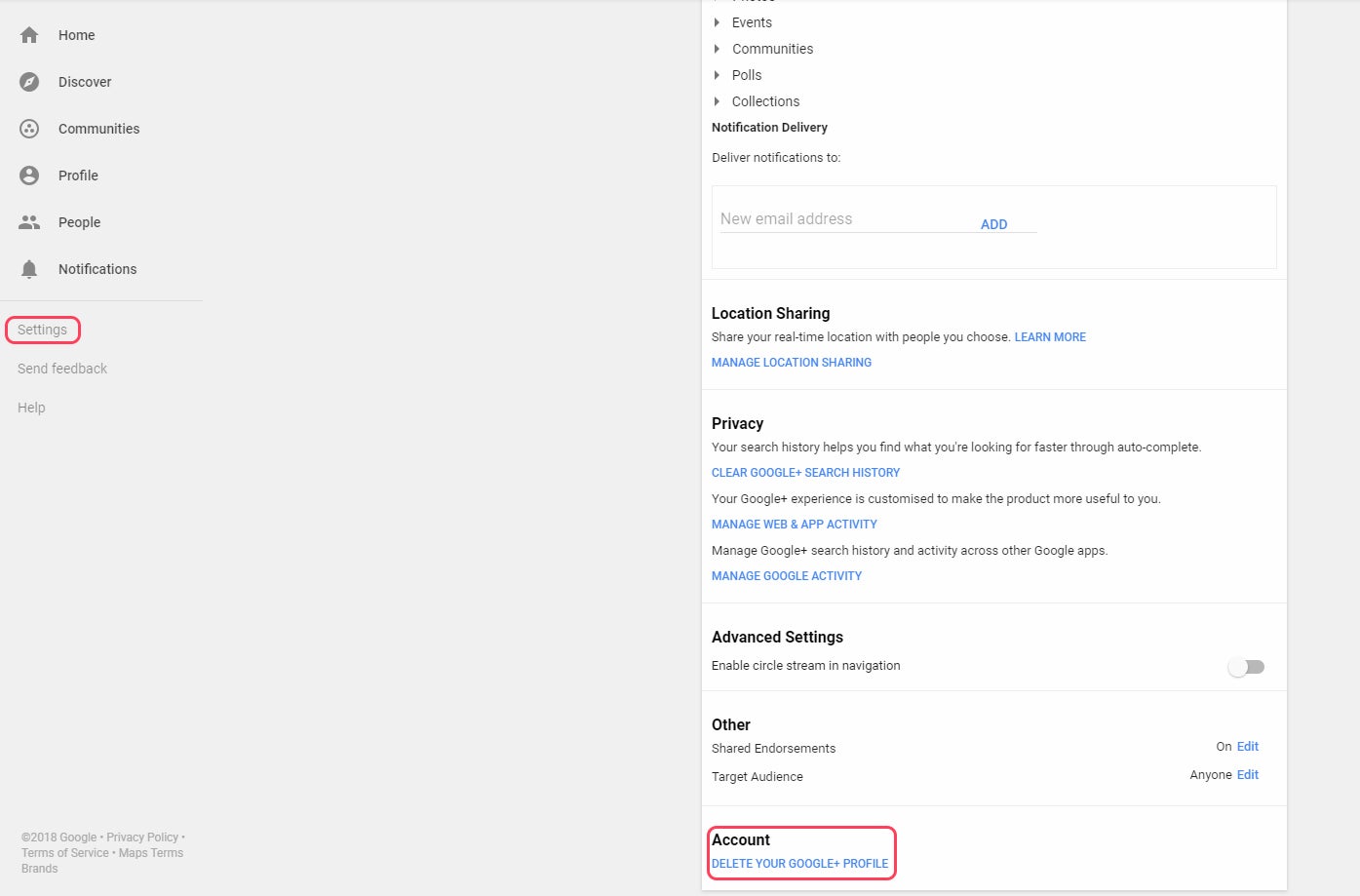This detailed screenshot captures a segment of Google settings, focusing particularly on viewing profiles. On the left side, there's a narrowly defined menu panel listing several options including Home, Discover, Communities, Profile, People, Notifications, and, separated by a thin divider, Settings, Send Feedback, and Help. Noteworthy here is the "Settings" option, which is specifically highlighted with a red outline.

Within the primary display, a seemingly expandable or pop-up panel provides intricate settings options, such as Add a new email address, Location Sharing, Privacy, Advanced Settings, Other, and Account. Of particular emphasis, given its own red outline, is the “Delete your Google profile” option, conspicuously marked in blue text at the bottom of this panel.

The overall screen suggests this might be an instructional guide, perhaps illustrating steps for deleting a Google profile. The red outlines draw attention to the crucial selections within the settings menu. It appears you would navigate to the Settings section and then scroll down within the overlay to find the “Delete your Google profile” option, which is positioned at the very bottom and likely indicates comprehensive account management details. The lower portion of the screen displays the copyright information, including "Copyright 2018, Google," followed by the Privacy Policy, Terms of Service, Map Terms, and Brands.